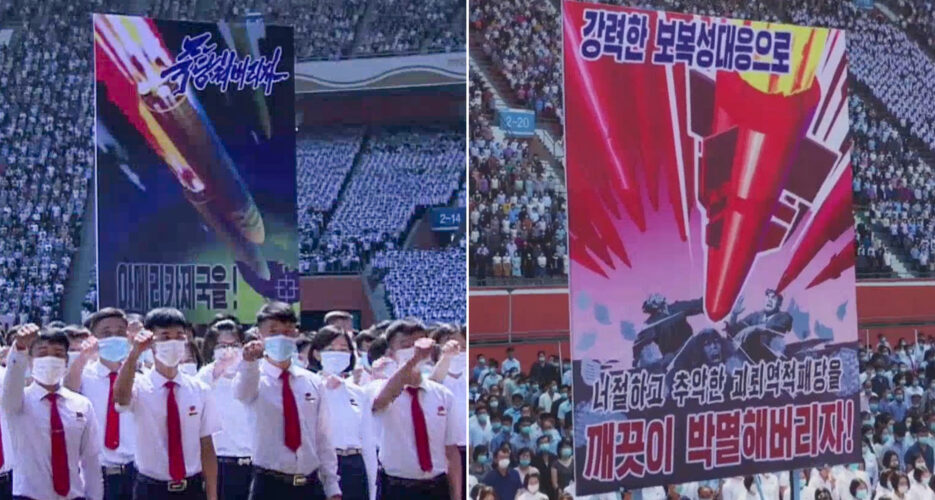The two side-by-side images depict a chilling scene in a large stadium, seemingly during a controversial rally. On the left, rows of young people, likely college-aged, are uniformly dressed in white shirts, red ties, black pants, and belts with small buckles. Each attendee wears a mask—some pink, some blue—and holds their right hand up to ear level in a fist. They all bear an emblem on their shirts that is indistinct, hinting at an organized uniformity. 

The backdrop features a prominent poster with vivid, colorful illustrations of bombs descending from the sky, accompanied by Asian characters, possibly Japanese or Chinese. The overall aesthetic and atmosphere suggest a militant communist gathering, seemingly celebrating weaponry.

On the right, a close-up shot emphasizes one of the banners amid the multitude of masked individuals in the stadium's expansive seating. The banner mirrors the left image with its depiction of bombs and vibrant Asian script, reinforcing an unsettling glorification of warfare and weaponry. The overwhelming visual impact of the masses and the militaristic iconography creates an eerie sense of indoctrination and power.